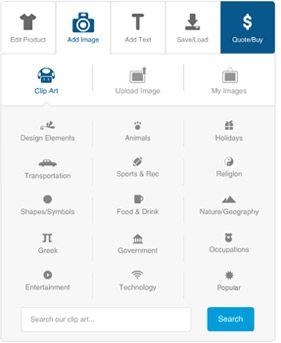A screenshot captured from a mobile device, displaying a user interface of a graphic design application. The navigation buttons are block-shaped and icon-based, typical of mobile app design. Despite the low image quality resulting in blurry graphics, the interface features a grey, blue, and white color scheme.

At the top of the screen, there are five key function buttons: 
1. "Edit Product" with a T-shirt icon 
2. "Add Image" with a camera icon 
3. "Add Text" with a T-icon 
4. "Save/Load" with a downward-pointing arrow icon 
5. "Quote/Buy" with a dollar sign icon.

Below these, three additional functional squares are present: 
1. "Clip Art" 
2. "Upload Image" 
3. "My Images."

Further down, a grey section contains 15 selectable icons representing various categories, such as Food & Drink, Technology, Religion, Animals, Transportation, and Shapes & Symbols. At the very bottom of the screen, there is a search bar accompanied by a blue search button, allowing users to search for specific clip art.